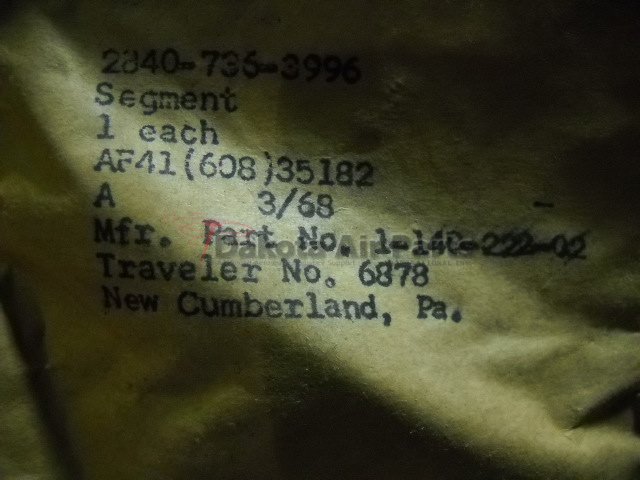In this image, we observe a highly blurred and darkened scene with muted colors, possibly depicting a portion of a label or paper. The overall indistinctness makes it challenging to discern specific elements, but there are noticeable contrasts between light and dark areas. A streak of light extends diagonally from the upper left to the lower right, accentuating the otherwise shadowy composition. The upper right corner of the image is particularly dark, approaching blackness.

Amidst the blur, we can distinguish black printed text in the center. The top line displays the numbers "2840736." Directly below, the word "segment" is visible. Continuing down, it reads "one each," followed by the alphanumeric sequence "AF4160835182." Further below, the text "MFR" appears, which stands for manufacturer, and its accompanying part number "1-140-220-02." Additionally, the phrase "traveler number 6878" is present, along with a reference to "New Cumberland, Pennsylvania."

This caption provides a detailed and structured description of the elements visible in the blurred image, emphasizing the mix of discernible printed text and obscured visual context.